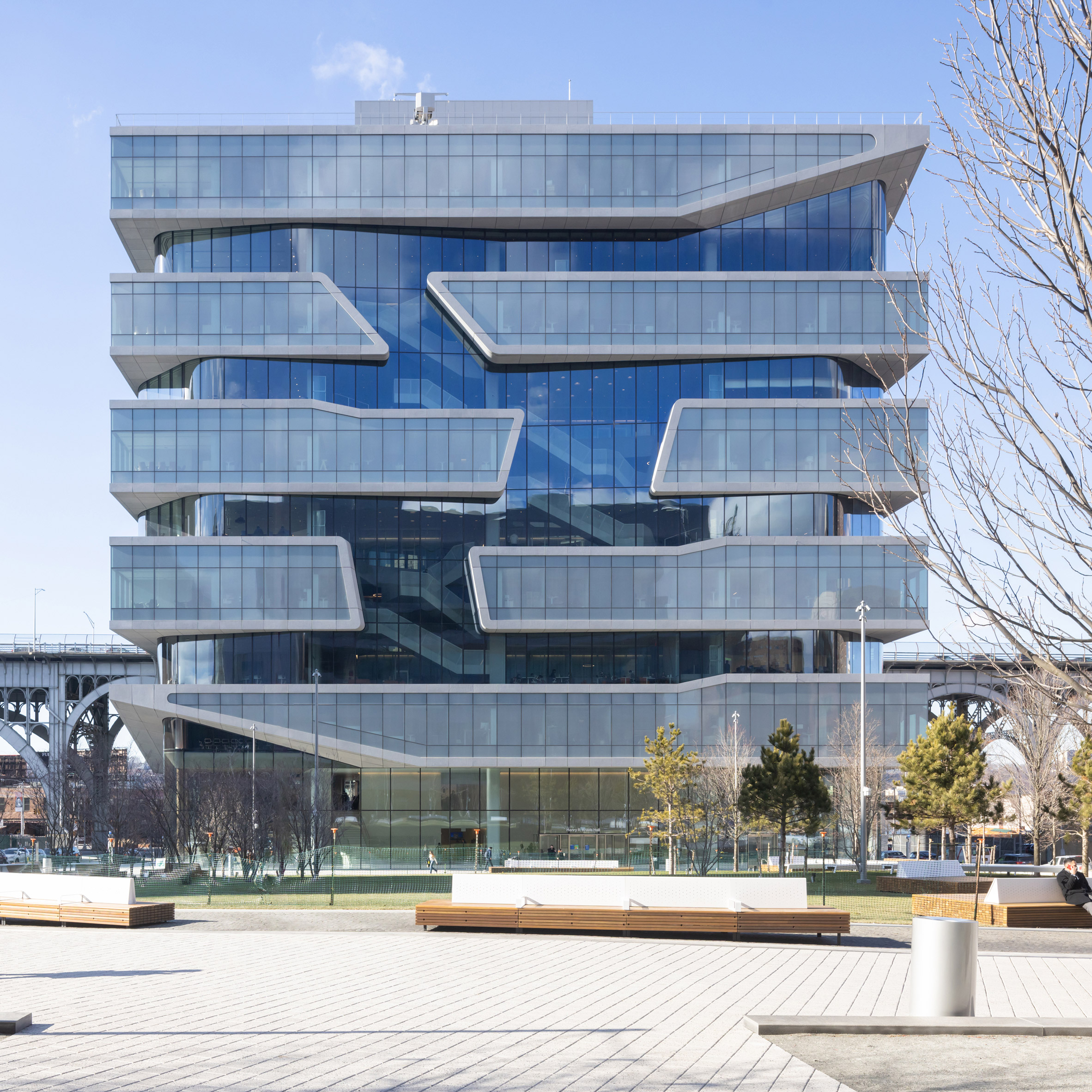This square image captures an innovative, five-story building with a striking, professional appearance. The building features a repetitive pattern of windowed sections framed by thick light gray borders, which visually distinguish the floors. Interspersed among these sections are recessed areas with flat, continuous glass panels, creating an interesting architectural rhythm that 'breaks off' and 'comes back together again,' while the overall structure maintains a square form. Dominated by a dark blue hue, possibly reflecting the sky or nearby elements, the building exudes a sophisticated blue-grayish tone. The ground level is adorned with a beige brick walkway, flanked by small, dark green and light green-leaved trees on the right and several leafless bushes or trees on the left. The backdrop showcases a mostly clear blue sky with a feathery white cloud hovering just above the building's left side. The photo meticulously captures the distinctive, glass-clad facade of the structure, illustrating its seamless blend of innovation and elegance in urban design.